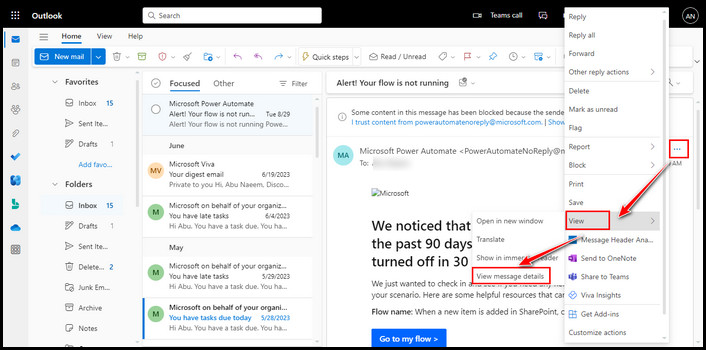The image showcases the user interface of an individual's Outlook email account webpage. 

In the top-left corner, the Outlook logo is prominently displayed. Adjacent to it, towards the right, lies a magnifying glass icon accompanied by a rectangular search box labeled "Search."

The far-left sidebar includes several navigational elements and folders:
- "Home"
- "View"
- "Help"
- "New Email"
- "Favorites"
- "Inbox 15"
- "Sent Items"
- "Drafts 1"
- "Add Favorite" (partially obscured)
- "Folders"
- "Inbox 15"
- "Drafts 1"
- "Sent Items" (partially obscured)
- Three periods indicating truncation for several folders such as "Deleted Items," "Junk Email," and "Archive"
- "Notes"

Directly to the right of the sidebar is another section with tabs labeled "Focused," which features a blue underline, and "Other." There is also a "Filter" option.

The "Focused" tab displays the following email summaries:
1. Email from "Microsoft Power Automate" with the alert "Your Flow Is Not Running" at 8:29, indicated by "... (ellipsis)"
2. Email from "Microsoft Viva" titled "Your Digest Email" with salutation, originally addressed to "Hi Abu Naeem" and partially cut-off message.
3. Email on behalf of the user’s organization, notifying the recipient "Hi Abu" about late tasks, dated 06/04/2023, with a partially visible message.

Beside this column, another detailed email is displayed:
- An alert notification from "Microsoft Power Automate" explaining that "Your Flow Is Not Running." The content provides information about past activities over 90 days and offers resources. The message is truncated but includes the Flow name "when a new item is added in SharePoint" and a "Go To My Flow" link.

The interface includes standard features for managing emails, making it subtly clear and navigable. The detailed structure signifies active engagement with the alerts and organizational updates from Microsoft services.